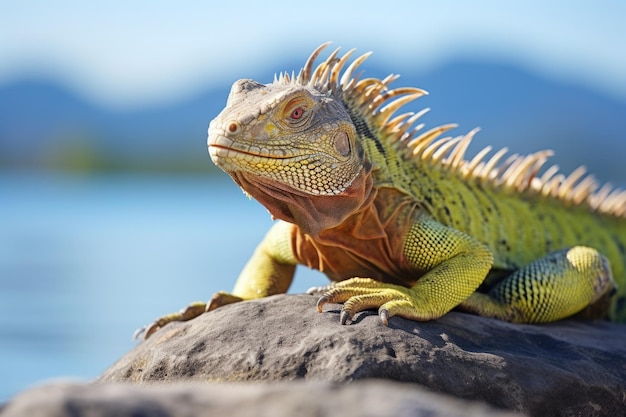The photograph captures a detailed scene featuring a vividly colored iguana perched on a gray rock, basking in the sunlight. The iguana’s body is a bright, neon green with a slight brownish tint to its head, and its underbelly and neck are characterized by wrinkly, orangish-brown skin. Sharp, beige spikes run along its spine from head to tail, adding an element of ruggedness. The iguana's scaly texture is visible on its arms, legs, and face, and it has dark, long talons on its claws. The animal’s eyes are red, with a distinctive look reminiscent of a dragon. The creature's mouth is closed, extending along its elongated face, and one of its nostrils features an orange dot. The iguana is looking left, with two prominent humps over its eyes at the front of its head. In the blurry background, a serene light blue body of water leads to a dark gray mountain range under a white sky. The entire scene is illuminated by sunlight, emphasizing the vibrant and contrasting colors of the iguana and its surroundings.